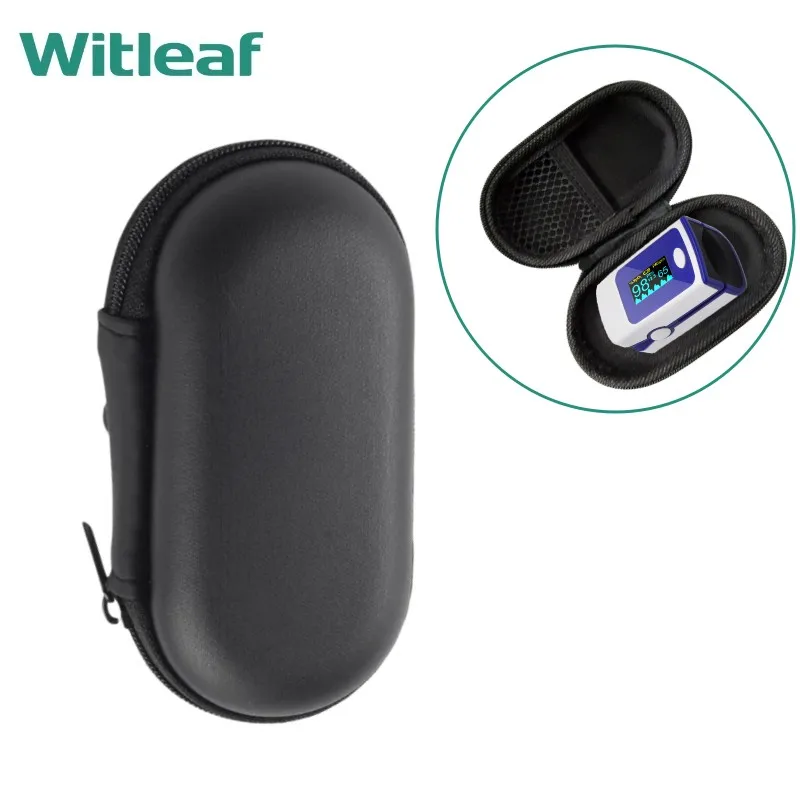The image features a high-quality color photograph on a clean, white background, resembling a retail product listing. In the top left corner, the logo "Whitleaf" is prominently displayed in bold, dark green lettering. The primary subject is a black, oval-shaped, hard-sided case with a zipper that runs around its center, making it look much like an eyeglass case.

To the right of the case, a circle outlined in bright green showcases the case in an open state, revealing its contents. The inside of the lid features a small mesh pocket, and the main compartment holds a compact, electronic monitoring device. This device is rectangular with a white and blue design and a digital display showing "98," suggesting it could be a pulse oximeter or similar health monitoring tool. The image is taken from a top-down perspective, providing a clear and detailed view of both the closed and open cases, accentuating the product's design and functionality.